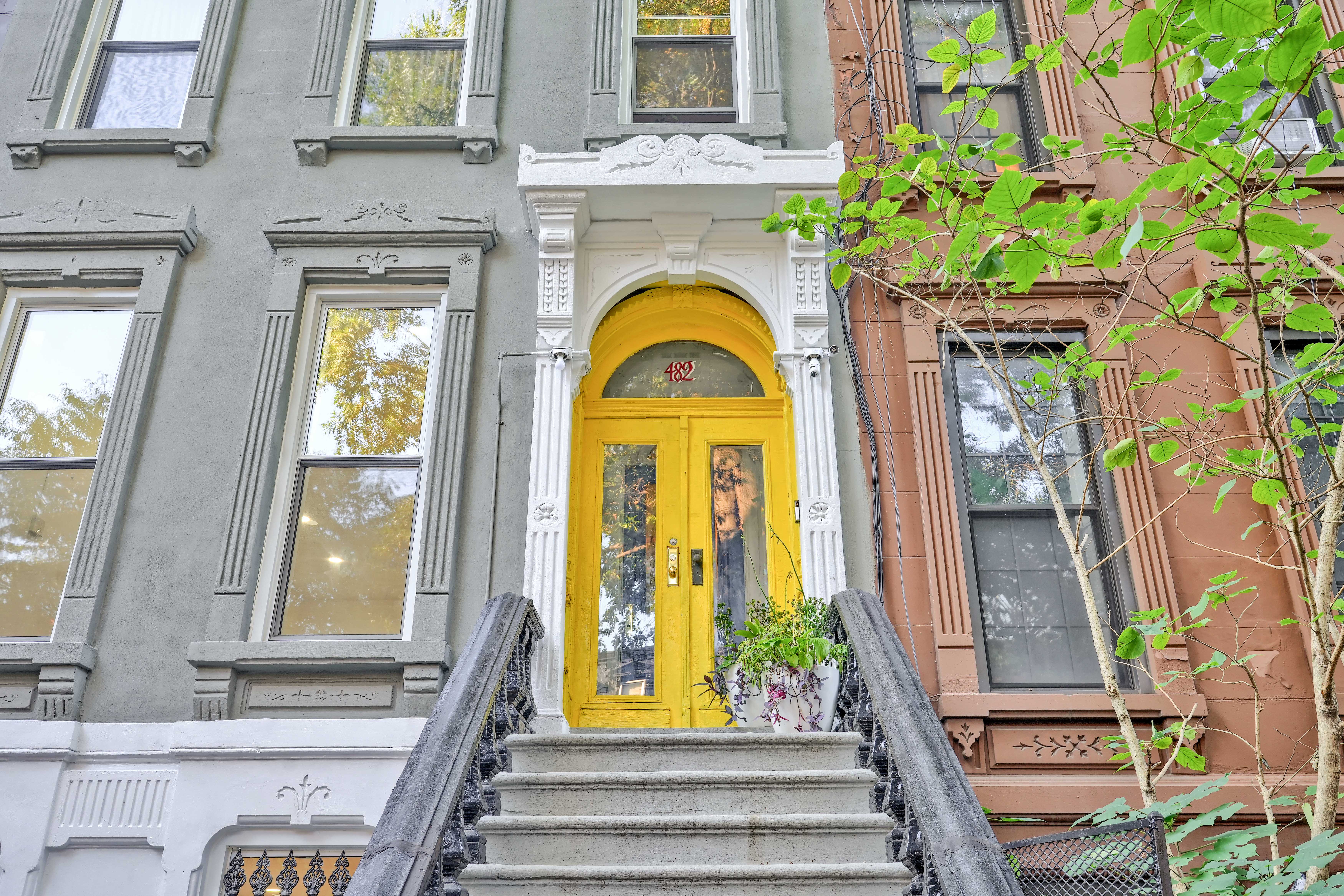This is a photorealistic image depicting the grand entrance of a building, possibly a row home or apartment on a city street. Taking up the entirety of the frame, the entrance features a set of steep stone steps leading up to a yellow double door with an arched top, framed by intricate white moldings. The solid yellow doors, marked with the number 482 in red, offer a striking contrast against the gray and brown facade of the building. The door handles and a doorbell are visible on the right. Just beyond the steps, we observe a large potted plant in a white planter, adding to the stately appearance. Surrounding the entryway, there are multiple tall windows with similar elaborate moldings, reflecting trees and the sky. There are five long windows positioned above the door and additional windows on either side, enhancing the building's symmetrical design. On the right side of the image, a small tree sapling with vibrant green leaves is visible, slightly obscuring the view. The right part of the building is clay-colored, featuring more windows and possibly a basement entrance, signified by the presence of gate-like structures below.